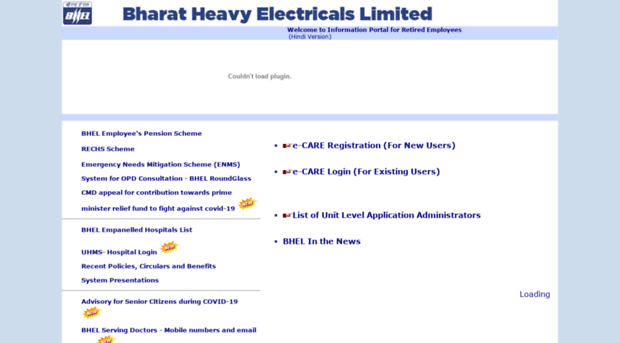The image depicts a website interface for Bharat Heavy Electricals Limited (BHEL), a company portal geared towards retired employees. 

**Background:**  
At the top left, there is a soft sky blue background tinged with a hint of gray, evocative of a pollution-affected sky. 

**Logo:**  
In the upper left corner, a white section contains the company's logo, which appears to read "B-N-E-L" or "B-H-E-L" in white text set against a blue background. Notably, the 'H' incorporates lightning bolt designs as its vertical elements, aligning with the full company name: Bharat Heavy Electricals Limited.

**Welcome Message:**  
Below the logo, a welcoming text states: “Welcome to your information portal for retired employees.”

**Main Banner:**  
Directly below the welcome message, there is a banner displaying an error message: "Couldn't load plugin," leaving this section blank and white.

**Information Section:**  
Underneath the banner, on another white background, smaller text lists multiple schemes and services related to BHEL:

- BHEL Employee Pension Scheme
- RECHS Scheme
- Emergency Needs Mitigation Scheme
- System for OPD Consultation
- BHEL Round Glass
- CMD Appeal for Contributions Towards Prime Minister Relief Fund to Fight Against COVID-19
- BHEL Impaneled Hospitals List
- UHMS Hospital Login
- Recent Policy Circulars
- Benefit System Presentations

**Advisory Section:**  
Following this, more detailed information includes an advisory for senior citizens during COVID-19, contact details for serving BHEL doctors including mobile numbers and emails.

**Right Panel:**  
On the right side of the page, four bulleted options are listed:
- e-Care Registration for New Users
- e-Care Login for Existing Users
- List of Unit Level Application Administrators
- BHEL in the News

Lastly, at the far right of the screen, there is a notice indicating "loading."

This comprehensive layout serves as a navigational guide and information hub for retired employees of BHEL, ensuring easy access to relevant schemes, contact information, and updates.